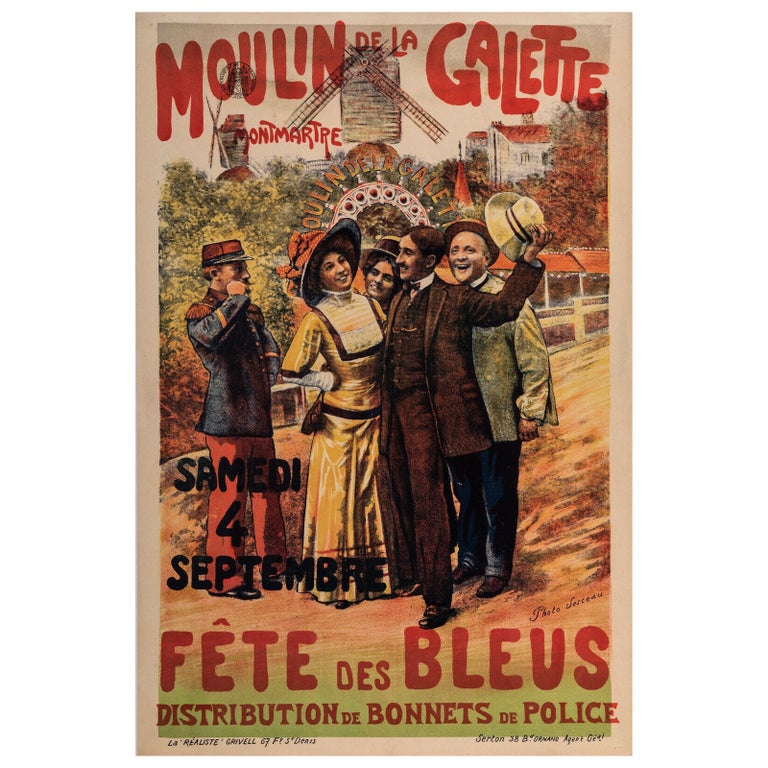This is an old advertisement poster, likely from the 1930s or 1940s, titled "Moulin de la Galette." The top of the poster features the text "Moulin de la Galette Montmartre" in a bold, red paint-like font, evoking a sense of nostalgia. The illustration depicts a lively, comic-like scene with five turn-of-the-century characters standing in the middle of a dirt road. To the left, a man dressed as an old-fashioned hotel concierge in a red top hat, red pants, and a blue jacket stands proudly. Next to him, a woman in a long yellow dress with a large hat adorned with a red ribbon embraces a man in a dark brown suit, who holds up a yellow top hat in his left hand. Just behind this couple, the head of another woman peeks into view, and to their right stands an old man. The background reveals a picturesque setting with trees, multiple windmills, and an arch sign, suggesting a cheerful festival atmosphere. The lower part of the poster includes the text "Fat Day's Blues" in red, followed by "Fete des Bleus" and "Distribution des Bonnettes de Police" in black, marking a festive and eventful occasion. The entire scene is set against a white backdrop, further enhancing the vivid colors and details of both the characters and their environment.